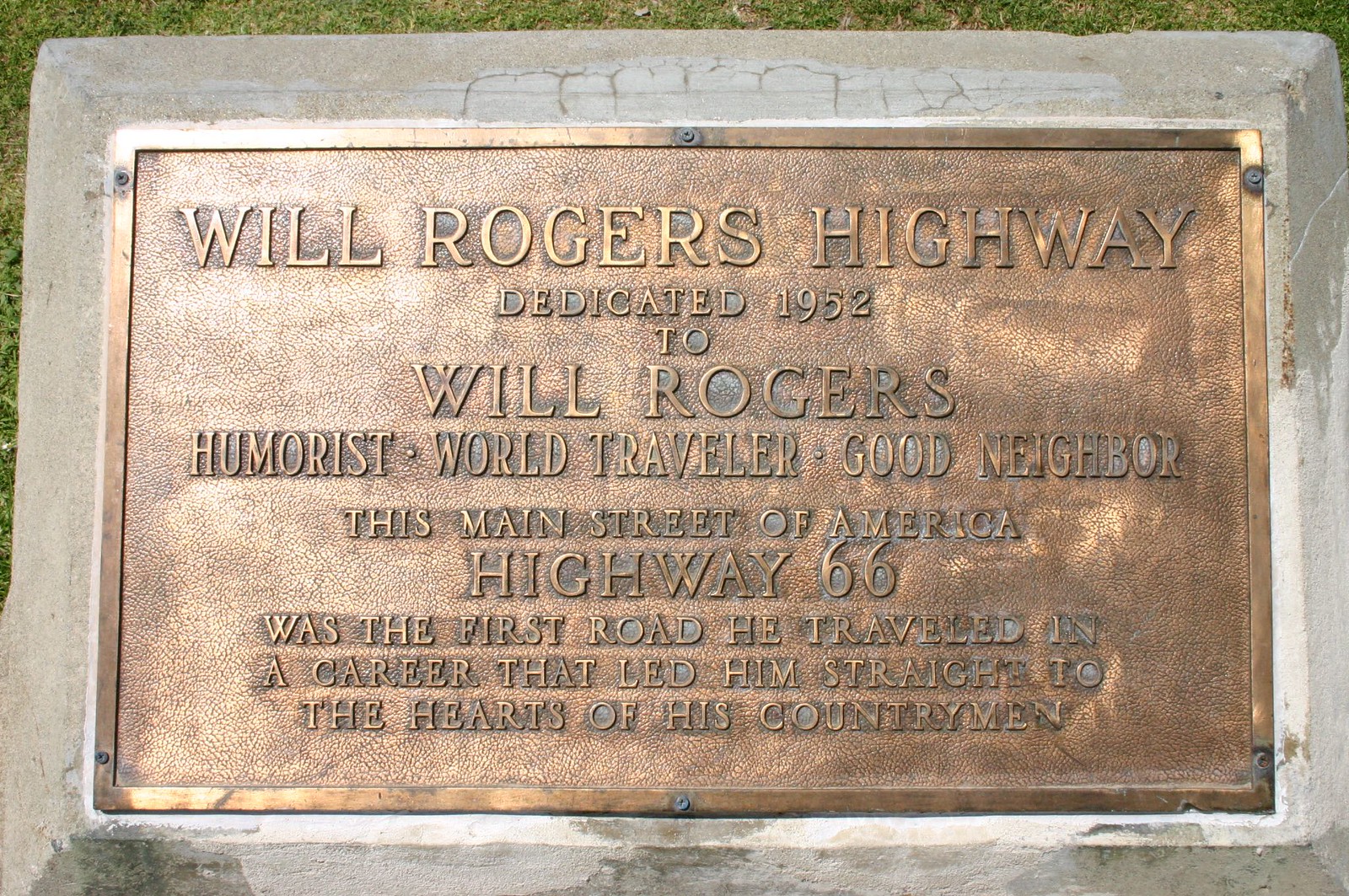The image depicts a commemorative plaque made of gold-colored metal attached to a gray and white stone base, which is likely concrete. The metal plaque, which is rectangular and somewhat tarnished with smudgy brown areas, is affixed with screws to the stone base. The surrounding area features patches of grass and greenery. The plaque reads: "Will Rogers Highway, dedicated 1952 to Will Rogers, humorist, world traveler, good neighbor. This main street of America, Highway 66, was the first road he traveled in a career that led him straight to the hearts of his countrymen". The text appears to be chiseled or pressed into the bronze-colored metal.